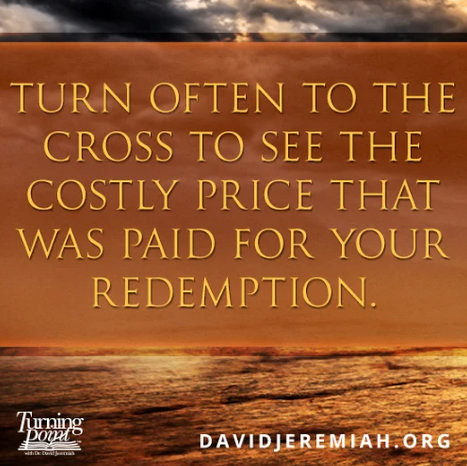This digital poster for Turning Point Ministries features a serene yet somber image background of an amber-tinted ocean and sky, transitioning from waves at the bottom to darker clouds at the top. Dominating the center of the image, in all caps and dark yellow text, is the inspirational message: "Turn often to the cross to see the costly price that was paid for your redemption." This message is set against a less opaque orange overlay, making the background more subdued. In the lower left-hand corner, there's a white logo featuring the name "Turning Point," with "Point" in italics and an open book outline beneath it. In the bottom right-hand corner, the URL "davidjeremiah.org" is prominently displayed, also in white. At the very top of the poster, a small section reveals a slightly blue sky with clouds, adding contrast to the predominantly amber scene.